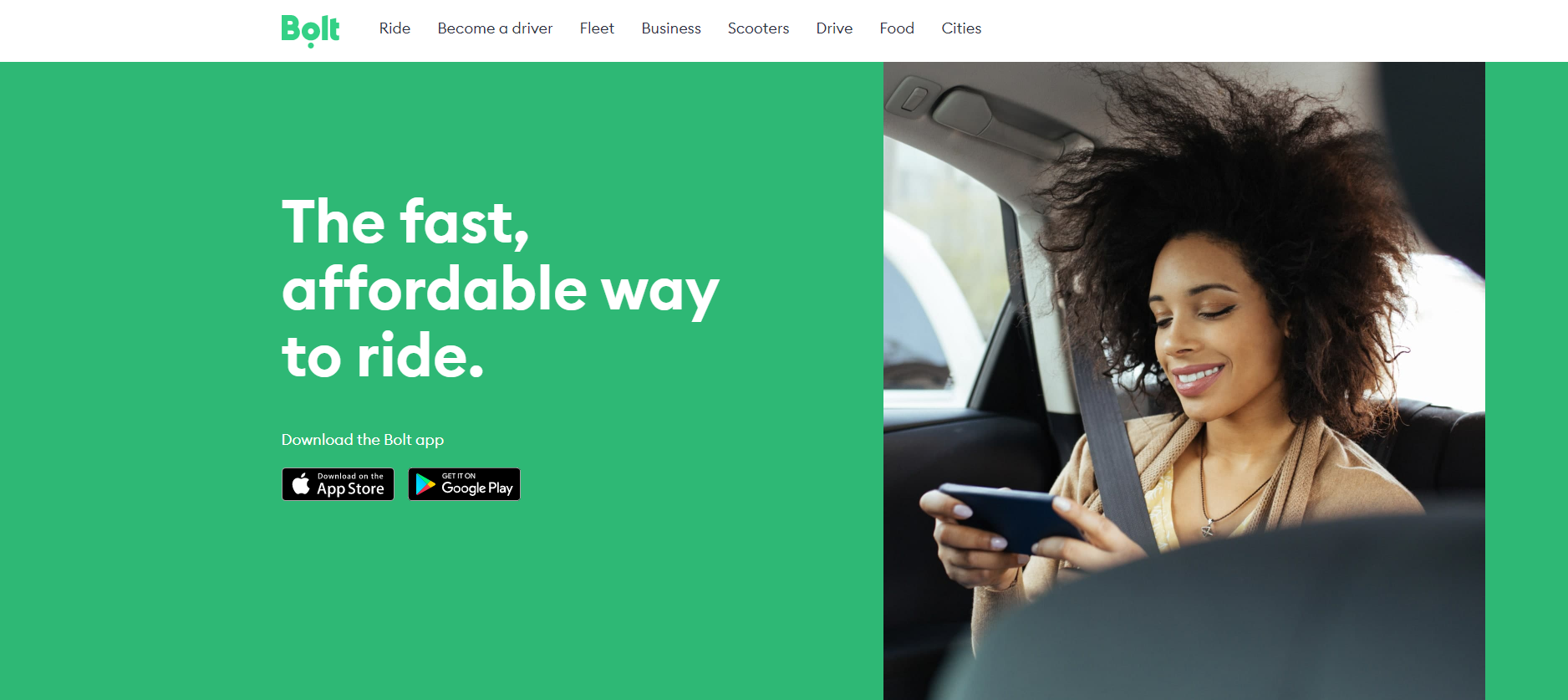The home page of the Bolt website is visually captivating with its predominant green color scheme. At the top, the Bolt logo is prominently displayed in green, accompanied by a navigation menu with options including "Ride," "Become a Driver," "Fleet," "Business," "Scooters," "Drive," "Food," and "Cities." A central message on a green background reads, "The fast, affordable way to ride," in white text, urging visitors to download the Bolt app. Icons for downloading the app from the Apple App Store and Google Play are prominently featured.

The main image shows a woman seated in the back of a car, securely fastened with a seatbelt. She is smiling as she looks at her phone, clearly enjoying her ride. Outside the car window, there is a glimpse of a white vehicle, suggesting that they are on the road, possibly a highway. This scene conveys a pleasant and safe riding experience.

Overall, the webpage has a clean, user-friendly design with white text and black clickable buttons, making navigation straightforward. This landing page effectively communicates Bolt's convenience and affordability to potential users.